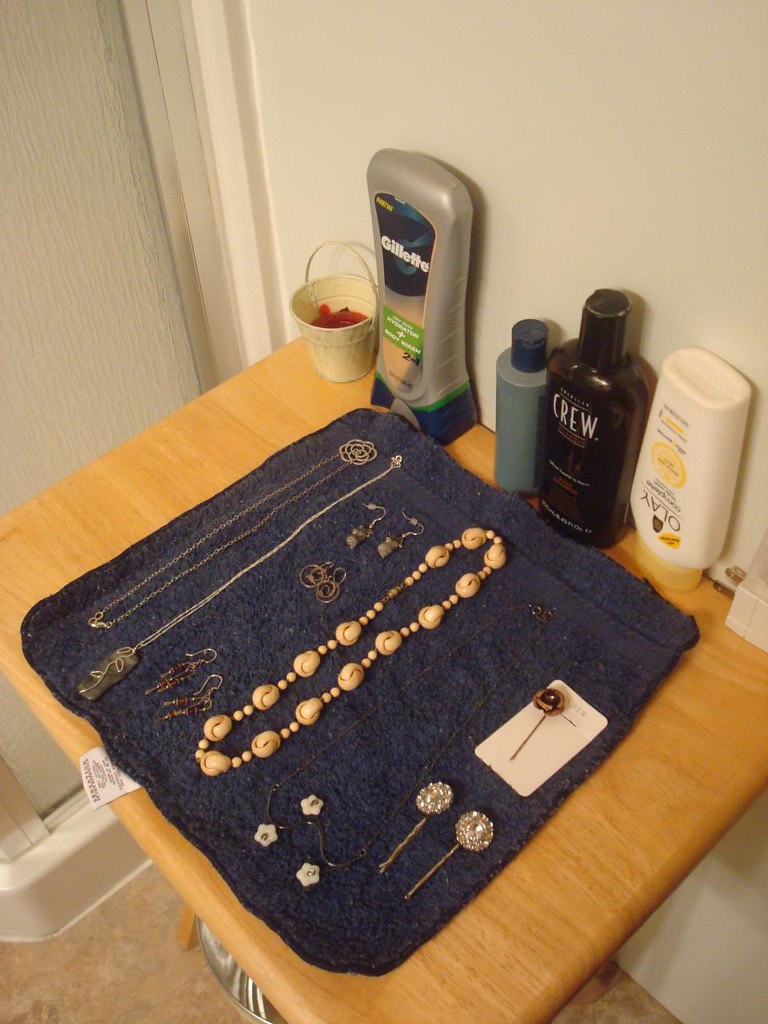In this image, we are presented with a detailed view of a bathroom corner. On the upper left, part of a narrow, crinkled-glass shower door provides privacy while revealing a hint of the shower area. The door has a white frame at its base which runs along the perimeter. Adjacent to the shower, on the right, is a small snack table with a natural wood stain. 

On top of the table lies a neatly spread white washcloth, showcasing an array of female jewelry and hair accessories. From left to right, the items include a flower-shaped necklace, a silver necklace with a leaf-engraved stone, three pairs of earrings made from wire, and a beige beaded necklace. Additionally, there are two identical circular barrettes with a crystal center, and a pin-like barrette adorned with a brown flower.

Leaning against the back wall of the table, thought to be the bathroom wall, are three bottles: a can of Gillette shaving cream, a black J.Crew product, and a white Oil of Olay bottle with a yellow cap. Also on the table is a small, tiny pail containing some red objects, adding a burst of color to the otherwise neutral-toned scene. This vivid arrangement presents a glimpse into a cozy and personal bathroom space.